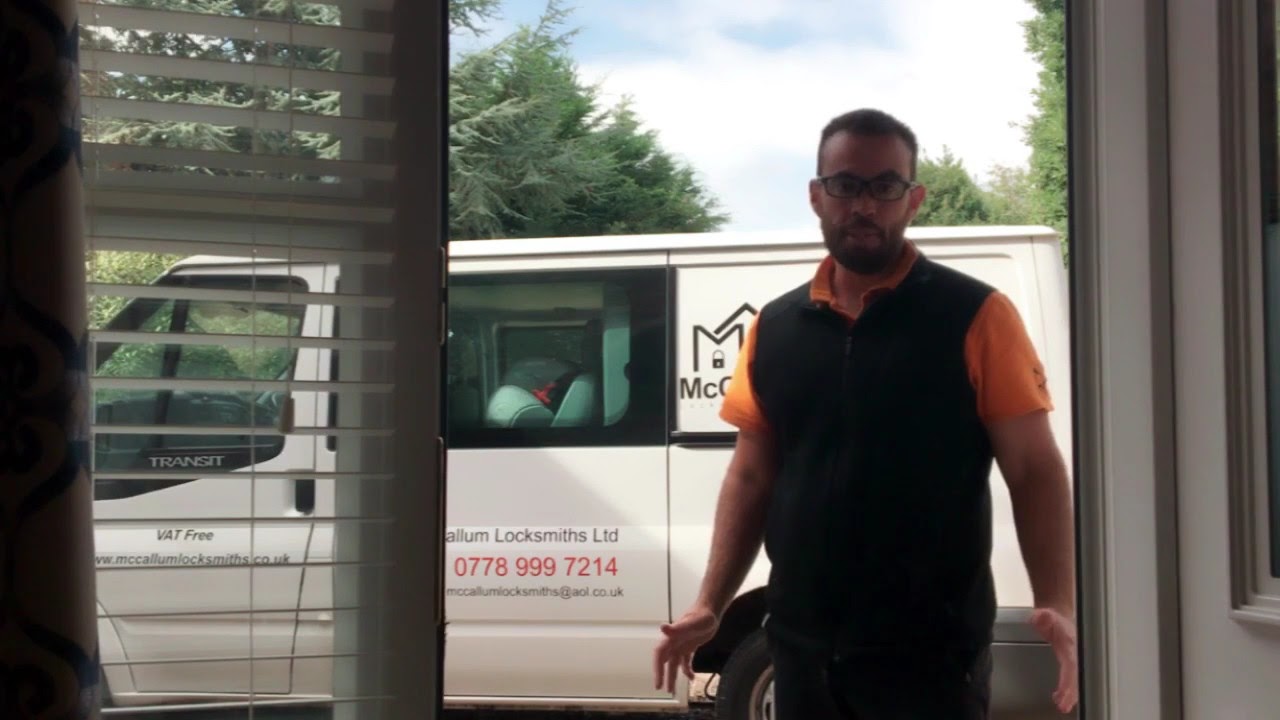The image depicts a sunny day with patches of clouds in a blue sky, casting natural light over the scene. Green trees provide a lush backdrop. A man with light skin is standing in front of an open doorway, partially obscuring it. He has black glasses and a black beard, and he is dressed in an orange short-sleeved t-shirt under a black, sleeveless sweatshirt with a zipper. The man stands facing the camera, suggesting he is aware of being photographed. 

Behind him is a white van, positioned with its front facing left. The van has an advertisement for a locksmith company with "Locksmiths LTD" written in black font and the phone number "0778-999-7214" in red font on the door. Additional black text, potentially including "VAT free" and a website, is also visible on the van. Part of a house icon is slightly visible behind the man, who obstructs most of the logo. Through the window beside the door, a set of blinds and a portion of a curtain with a blue design can be seen, indicating an indoor space adjacent to the man’s position.